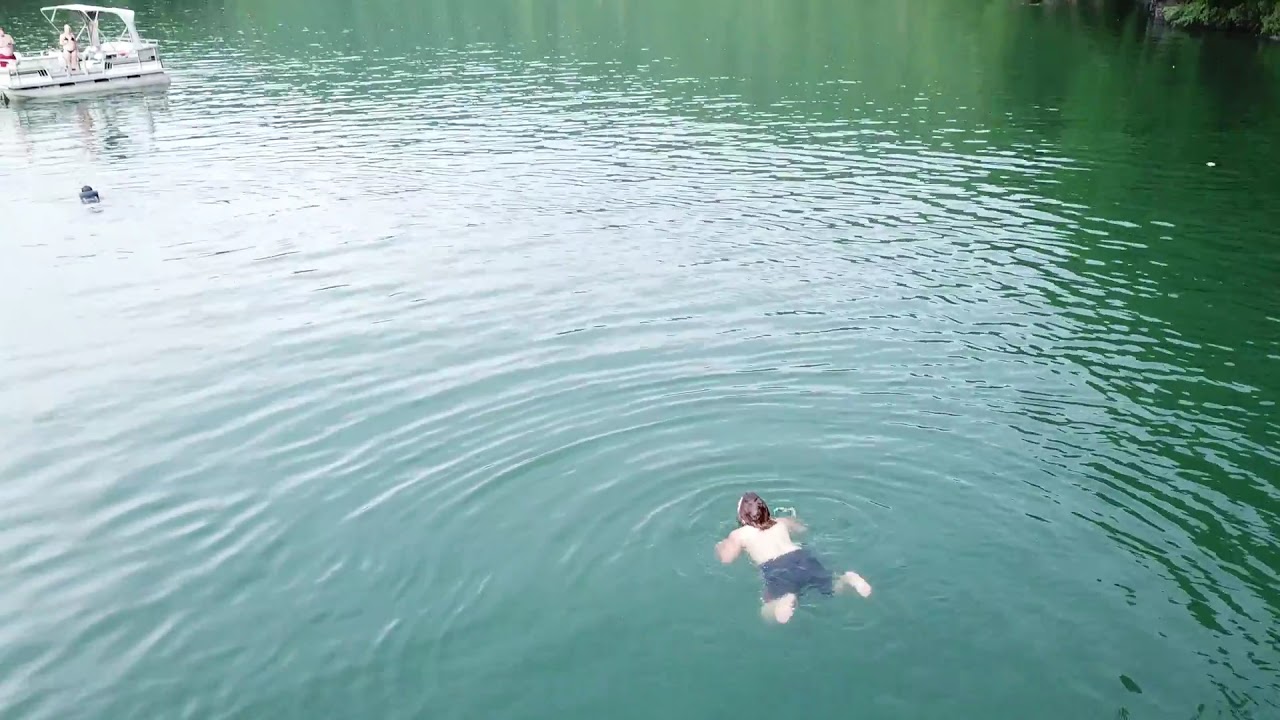In this daytime image, a person is swimming in a serene, green lake. The swimmer, a light-skinned male with wet brown hair, is wearing dark blue swim trunks and appears to be performing the butterfly stroke, with his arms and legs tucked in, preparing to extend outward. The lake water, varying from dark green to an emerald green with a bluish cast, reflects a lot of light, making it difficult to discern its true color. The swimmer is positioned in the lower right corner, moving towards the upper right corner, where the water lightens due to sunlight. In the top left corner, partially obscured by greenery, a small white boat is visible, approximately 50 feet away from the swimmer. The boat, capable of holding about six people, has at least two individuals on board, a man in swim trunks and a woman in a bikini, both observing the swimmer. The scene is calm and serene, filled with gentle ripples in the water.